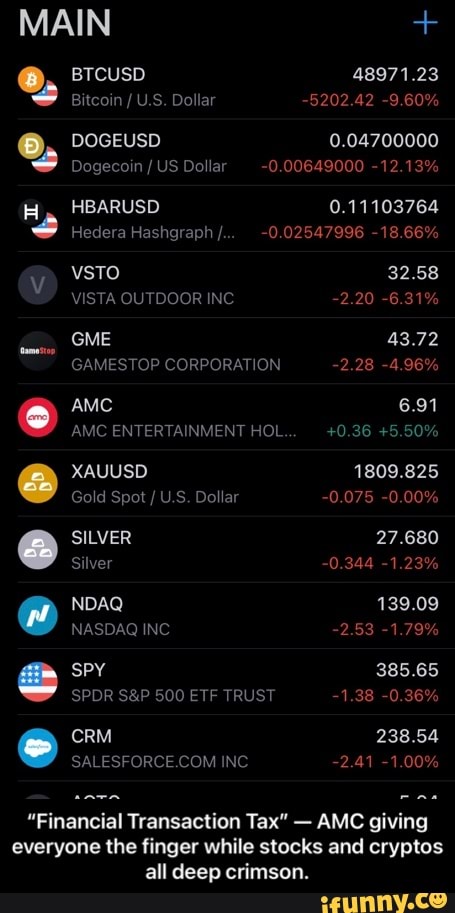A screenshot from a cell phone displays a predominantly black interface with various elements and text. At the top left corner, in bold, capital letters, is the word "MAIN," while on the top right corner, a plus sign is visible. Along the left side of the screen, there is a vertical column of icons. Adjacent to these icons, in the middle section, corresponding labels or descriptions are written. On the far right side, there is a column of numbers, with some additional numbers underneath. At the bottom of the screen, the text "FINANCIAL TRANSACTION TAX" is present. The caption mentions AMC's reaction to the market with "AMC giving everyone the finger while stocks and cryptos all deep crimson," followed by the watermark "IFUNNY.CO." At the top of the screen, two icons are shown side by side with the label "BTCUSD" and the value "48971.23," accompanied by two numbers underneath. This pattern of icons, labels, and numerical values repeats consistently down the length of the screen.